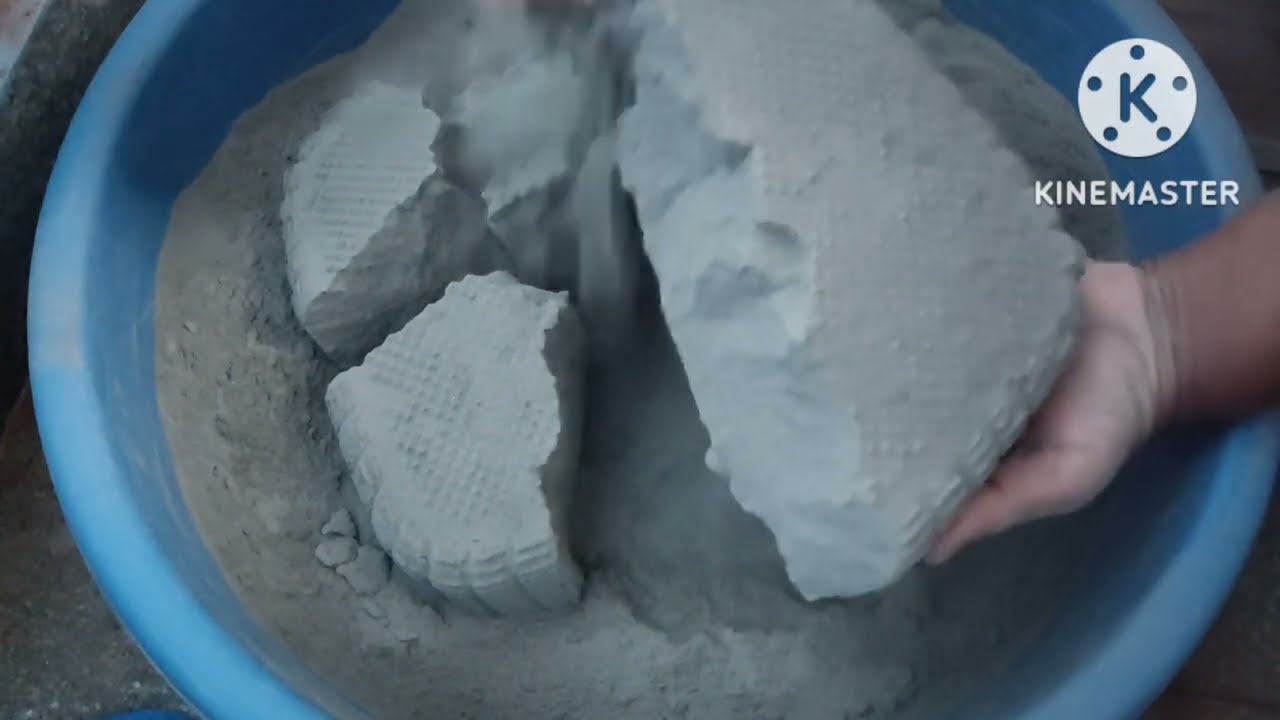The image depicts a close-up of a person’s hand reaching into a large, light blue flower pot or bucket filled with broken and crushed cement pieces, some of which appear as crumbled powder. The hand is holding a solid block of the cement, amidst an array of textures suggesting partially recycled or reused material. The cement, which ranges from solidified chunks to fine dust, indicates an ongoing project, possibly an art endeavor or a recycling effort. The scene is likely shot from a tutorial video on cement mixing, evidenced by the grainy quality of the image and a watermark in the upper right corner displaying the KineMaster logo – a white "K" encircled by five dots. The overall setup hints at a methodical process requiring time and effort to break down and reuse cement, with the light blue and gray tones dominating the visual frame.